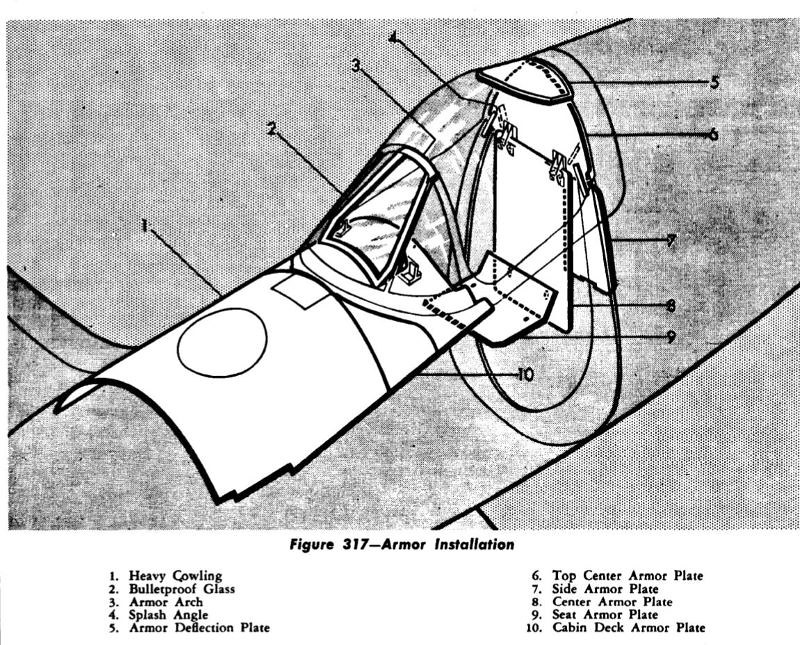This black-and-white sketch is a detailed drawing of an aircraft cockpit, specifically its armor installation. The image is rectangular, wider than it is tall, and depicts the seating area of what appears to be a single-person enclosed plane. The cockpit illustration prominently features a white background, while the surrounding areas utilize gray lines and muted tones. The sketch includes annotations with numbers 1 through 10, each pointing to different parts of the cockpit armor installation. Below the picture, a caption in black print reads "Figure 317 - Armor Installation," followed by a list that describes each numbered component: 1. heavy cowling, 2. bulletproof glass, 3. armor arch, 4. splash angle, 5. armor deflection plate, 6. top center armor plate, 7. side armor plate, 8. center armor plate, 9. seat armor plate, and 10. cabin deck armor plate. The list is neatly divided into two columns under the drawing, detailing the specific areas of armoring within the cockpit.